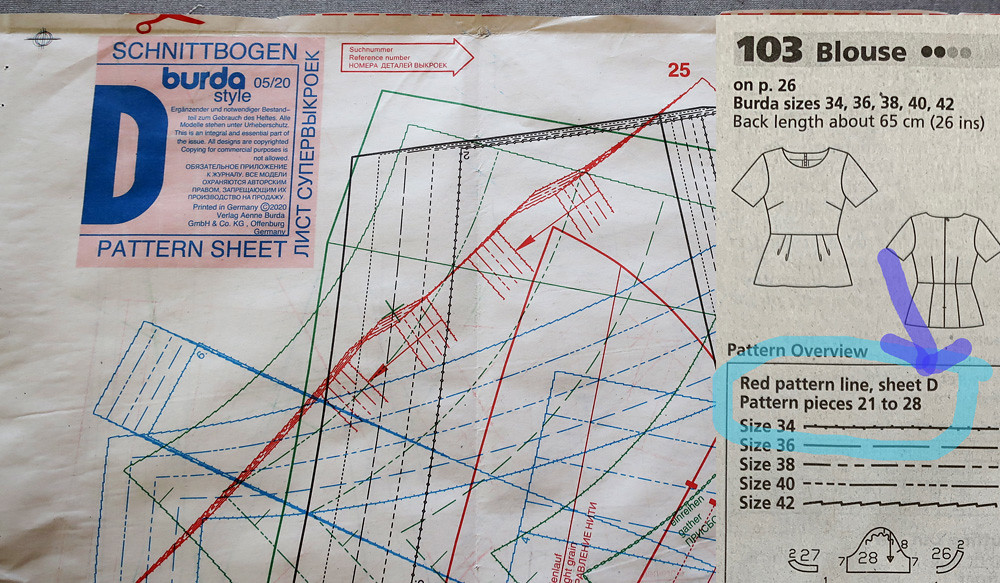The image features an intricate layout of what appears to be a detailed blueprint or pattern sheet for a blouse, centrally positioned and likely hung on a wall or placed on a table in an indoor arts and crafts room. At the top, the text "Schnitt-Bogen Bertha style pattern sheet" is prominently displayed. The blueprint illustrates a cutting pattern for a blouse, with the sizes specified as 34, 36, 38, 40, and 42. Detailed directions and pattern lines are marked in multiple colors including gray, white, blue, pink, red, dark blue, and purple.

On the upper left corner, there is a pink box containing various texts. It includes "Berda style 05/20" along with "Printed in Germany C2020" and additional cautions about copying designs for commercial purposes. Surrounding these texts, there are various words in different languages, including Russian and German.

To the right, a vertical light gray box lists further details about the "103 blouse" with pertinent measurements like a back length of 65 centimeters (26 inches). It includes front and back illustrations of the blouse, a pattern overview circled in blue, and directions indicated by a purple arrow. The various sizes are represented by distinct line designs, with pattern pieces numbered from 21 to 28. The blueprint is adorned with numerous thin lines and directional arrows in multiple colors such as green, blue, red, and black.